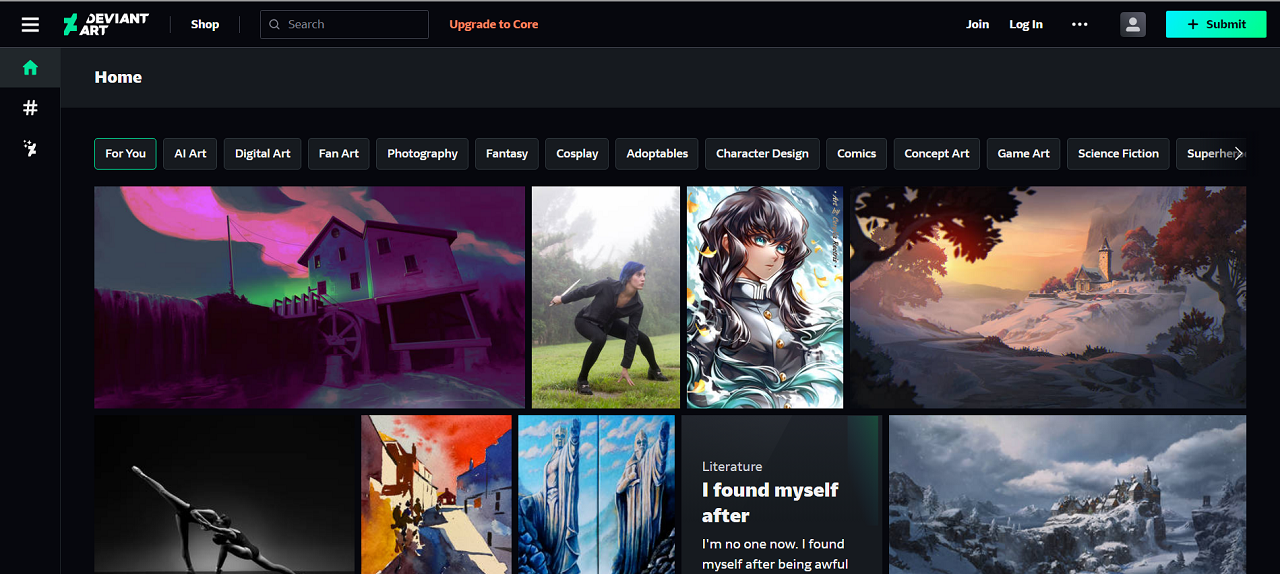This image showcases the homepage of the website deviantART. At the top of the page, the word "deviantART" is prominently displayed in black, accompanied by its intricate logo on the side. Adjacent to these, there are various navigational tabs: "Home," a tab marked as "dubber," and another featuring the deviantART logo.

The primary section of the website interface features multiple tabs organized horizontally. The currently active tab, indicated by a green outline, is labeled "For You." Following it, there are several other tabs with categories such as "AI Art," "Digital Art," "Fan Art," "Photography," "Fantasy," "Cosplay," "Adoptables," "Character Design," "Comics," "Concept Art," "Game Art," "Science Fiction," and "Super Hero." Notably, the "O" in "Super Hero" appears to be slightly cut off.

Below these tabs, a collection of nine images is displayed. The top row consists of four large landscape pictures, with two prominent images on each side. Following this, several other smaller pictures are arranged, filling the content area below the tabs.